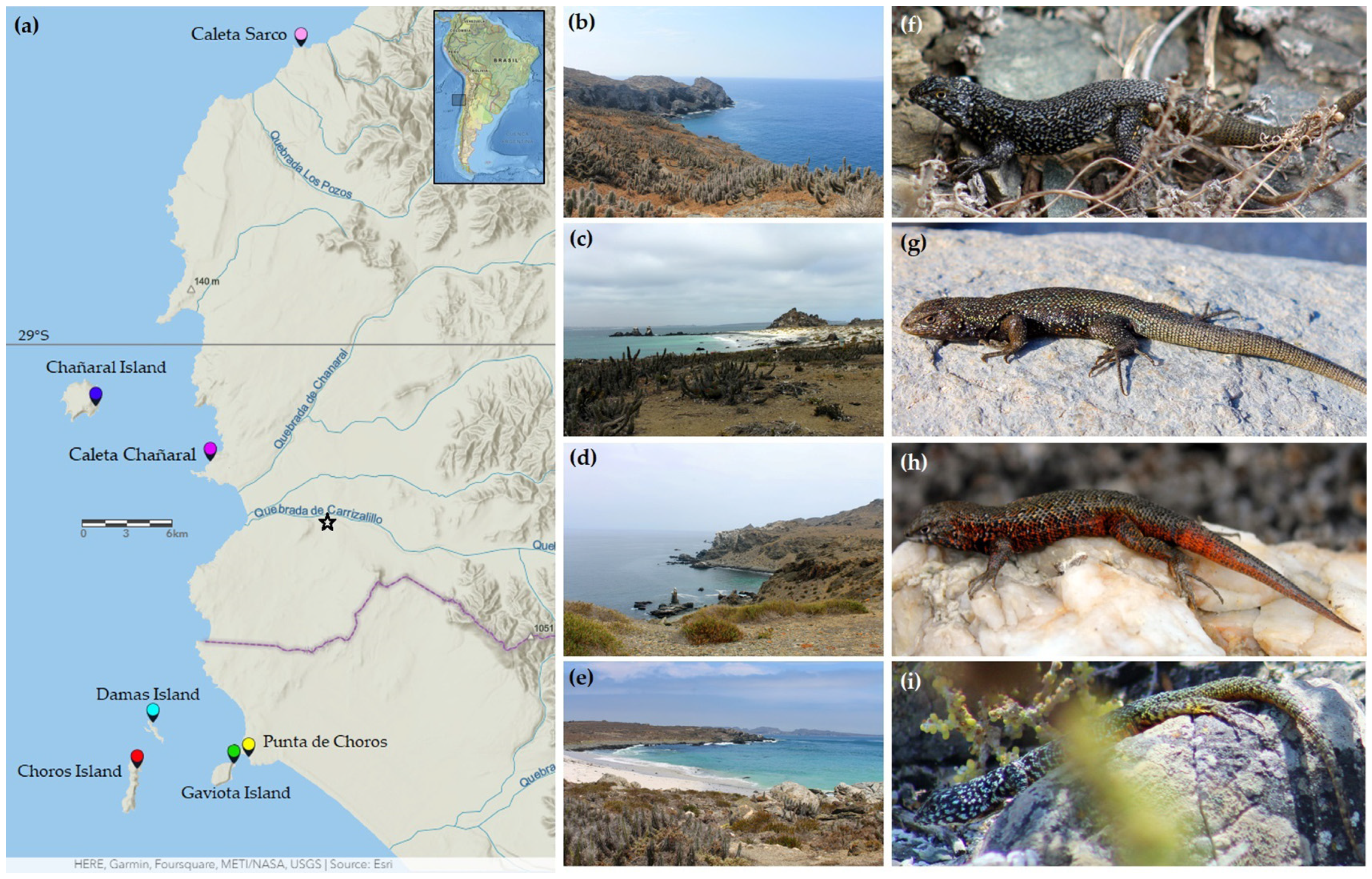The image is a detailed collage comprised of several photographs and a map, likely highlighting a coastal region in South America near Chile. On the left side, there is a vertical rectangle map presenting the area with blue indicating water on the left and a gray landform on the right. This map is labeled with various geographic markers, including Colecto Sarco at the top, and Colecta Shannaral and Shannaral Island on the left. At the bottom, different colored dots indicate Damas Island, Coros Island, Punta de Coros, and Gaviota Island.

On the right side, the collage features two sets of labeled photographs. The first set (B, C, D, and E) showcases landforms surrounded by water, with B, C, and D depicting verdant landscapes and E marked by exceptionally clear water. The second set (F, G, H, and I) displays various lizards atop rocks, each with distinct coloration: a black lizard at the top, followed by a greenish one, then one with a reddish tint, and finally a blue and yellow lizard. The overall collage paints a vivid picture of the local environment, highlighting both the natural landscapes and the fauna native to this coastal area.